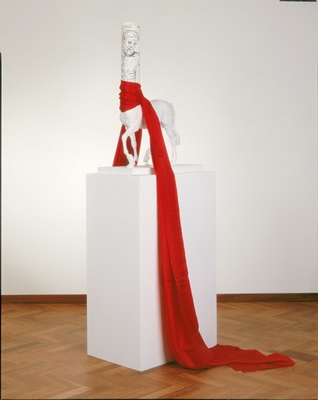The photograph showcases a highly detailed white centaur sculpture, prominently displayed in what appears to be a museum or art gallery. This intriguing piece of art combines the torso and head of a man seamlessly with the body and legs of a horse. The man's torso, fashioned in a more simplistic and flat style, contrasts with the meticulously crafted horse's body, which features an elevated leg. A vivid red cloth strikingly wraps around the intersection of the two forms, draping gracefully over the rectangular white pedestal and extending down to the brown wooden floor. The floor beneath the stand consists of a mix of dark and light brown wood panels arranged in a zigzag pattern. In the background, a white wall is intercepted by a brown wooden bar, providing a clean separation between the floor and the wall, highlighting the statue's placement and adding to the gallery's tranquil ambiance.